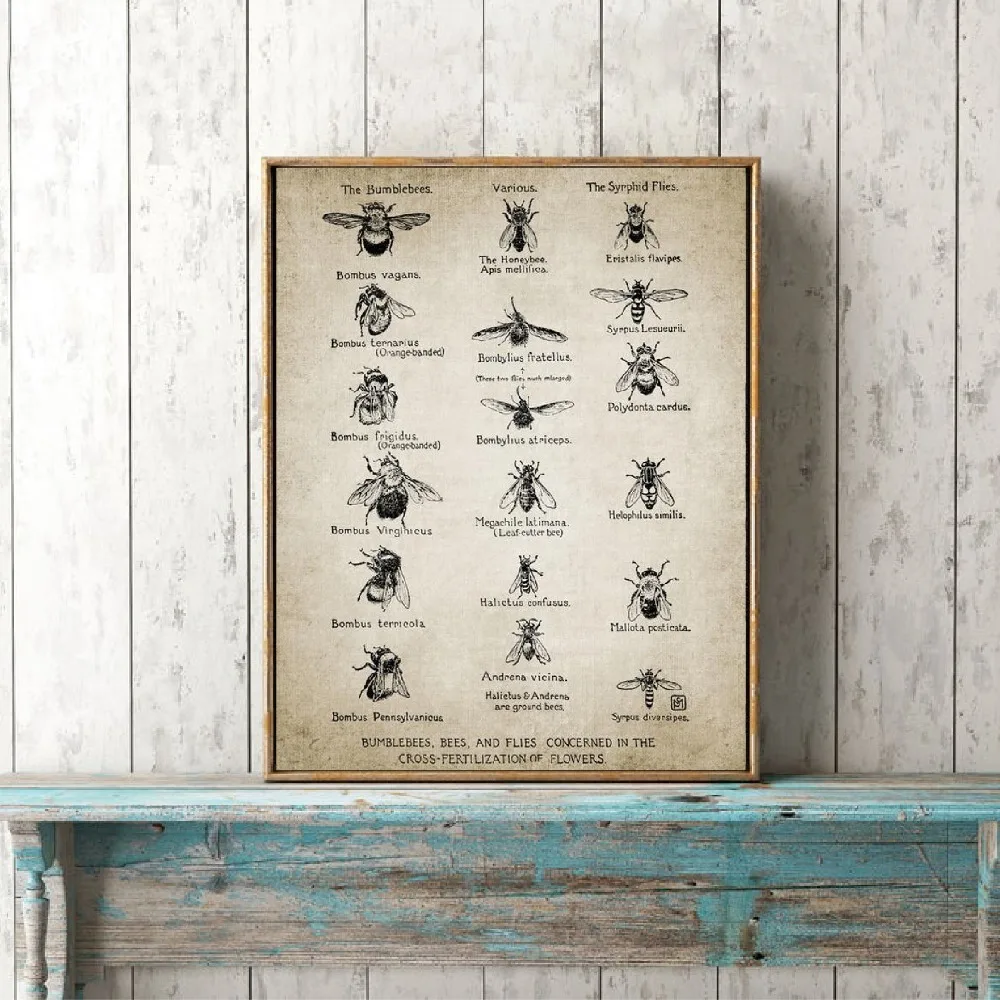The image is a square-shaped, realistic photograph framed by a thin, light-colored wooden border, measuring approximately 1.5 feet across and 2 feet tall. It is set against a weathered wooden wall with vertical white slats and an aged, blue-green painted horizontal shelf below. The framed picture inside shows a vintage-style illustration of 18 different insects, hand-drawn in black ink on a background resembling aged parchment, with a lighter center and darker edges. The insects are arranged in three vertical columns, each containing six rows. The left column features bumblebees, the middle column is labeled "various" and features different types of bees, and the right column depicts surfeit flies. Each insect is meticulously illustrated, with names annotated below each drawing in black text. At the bottom of the print, it reads "Bumblebees, bees, and flies concerned in the cross-fertilization of flowers," emphasizing the role of these insects in pollination. The overall setting and style suggest an old, distressed aesthetic, possibly within a vintage or rustic environment, like a museum or a historic home.